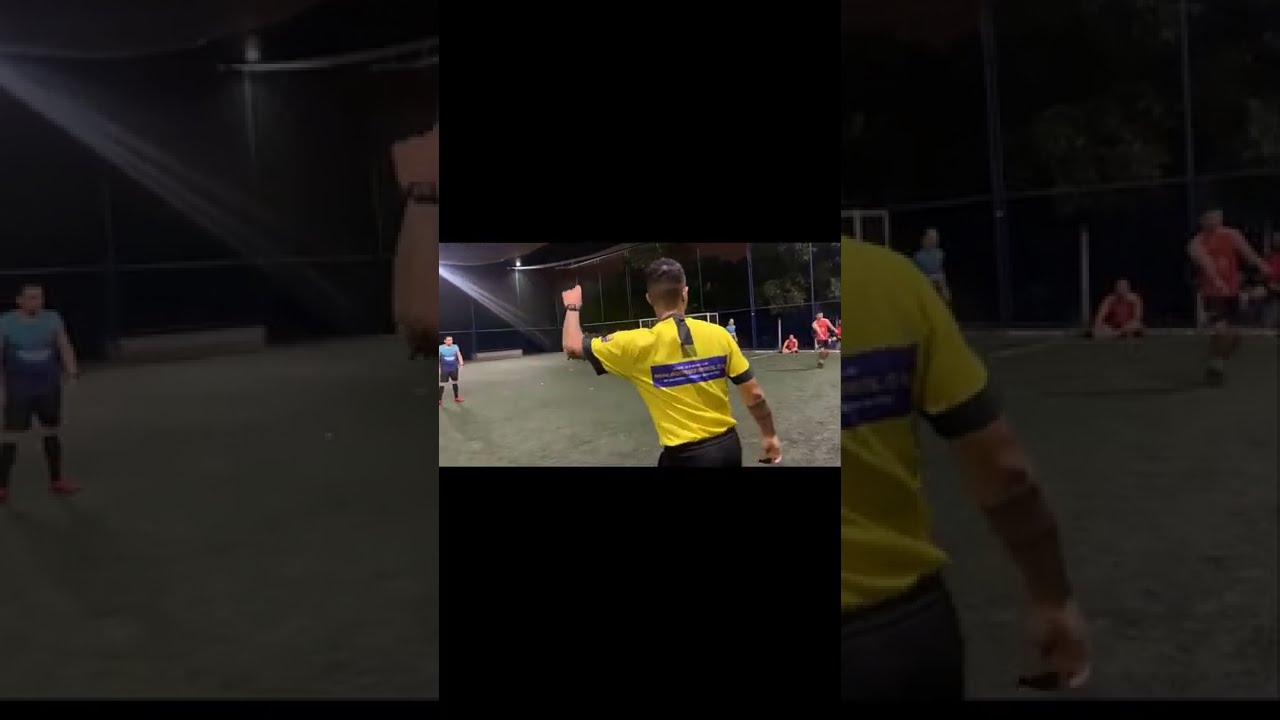A vertically taken photo captures a nighttime outdoor sports scene, illuminated by surrounding electric lights. The focus is on a man, presumably a referee, standing with his back to the camera. He wears a bright yellow jersey accented with blue and black, along with black shorts. His left arm is raised with his elbow bent, trying to call the attention of the players. The event takes place on a grassy field enclosed by long fences or netting. In the background, four or five other men, dressed in sports uniforms, which include red shirts, are either standing or moving on the court. The dark surroundings and the positioning of the players suggest an active and engaging match.